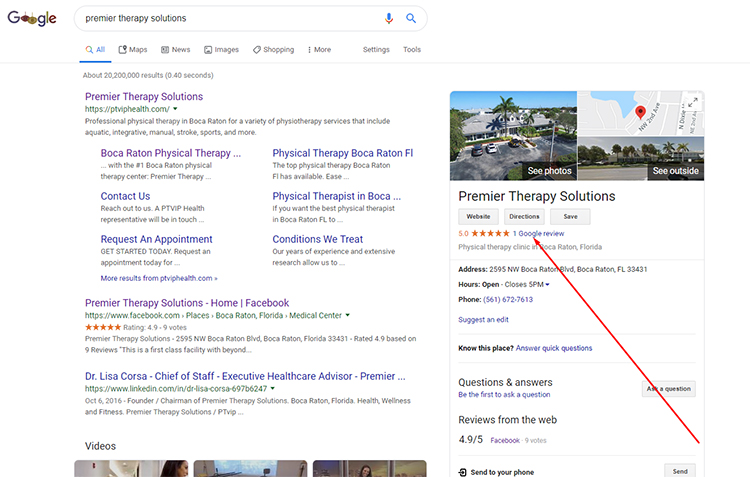The image depicts a Google search results page for "Premier Therapy Solutions." At the top, the Google logo is visible, with the two "O"s animated to resemble spinning tops. In the search bar, the query "Premier Therapy Solutions" has been entered. Below, the first search result link appears in purple, indicating it has been previously clicked. The link leads to information about Premier Therapy Solutions in Boca Raton, Florida, including sections such as "Contact Us," "Request an Appointment," "Physical Therapy," "Conditions We Treat," and mentions of Boca Raton Physical Therapy.

Further down the page, there is a link to their Facebook page and information about Dr. Lisa Corsa, the Chief of Staff. The bottom of the search results displays three videos related to the topic, but only their upper portions are visible.

On the right-hand side of the screen, there is an informative visual snippet about Premier Therapy Solutions. This snippet includes a photograph of their facility's exterior and a small map. Several interactive buttons are available, such as "See Outside," "Website," "Directions," "Save," and options to view their opening and closing hours along with their phone number. The snippet also highlights their five-star rating and a single Google review, emphasized by a red arrow pointing towards it.